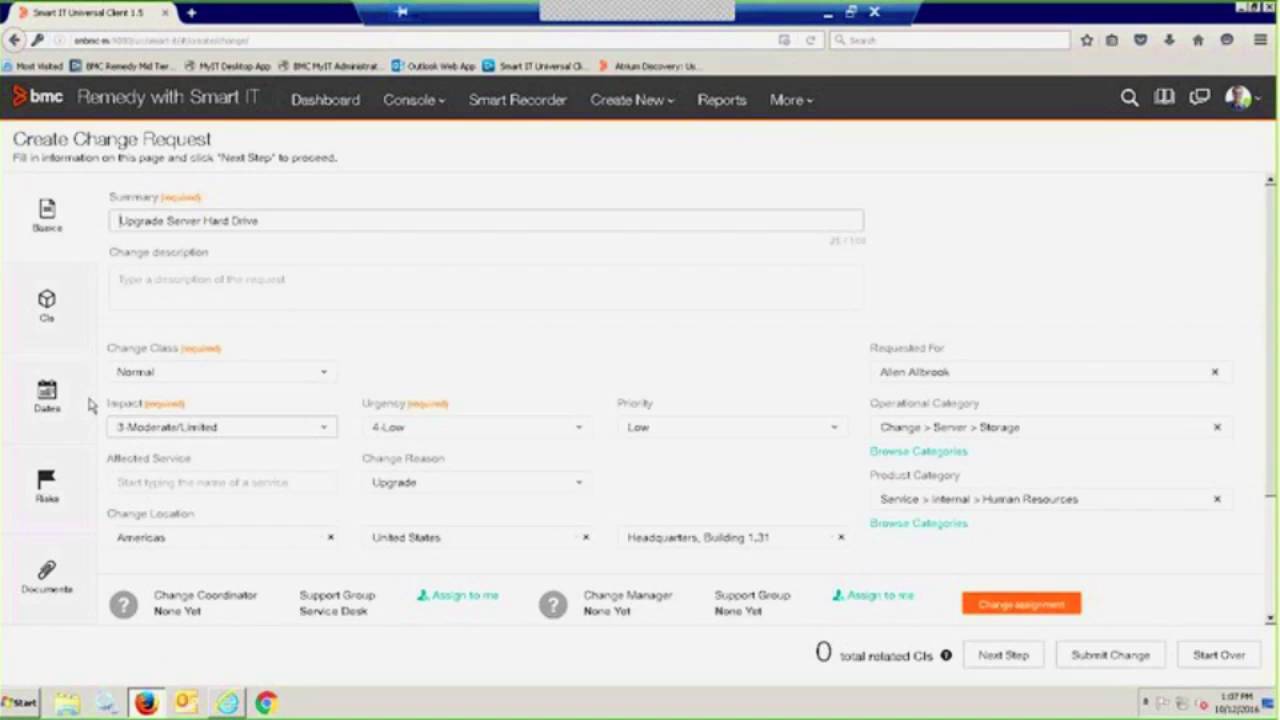This image showcases the BMC website interface. At the top, there is a long, dark gray header strip displaying the BMC logo prominently to the left in bold, bulky white lowercase letters. Adjacent to the logo, a slightly faded red design is present, although its details are hard to discern. To the right of the logo, the text "Remedy with Smart IT" is shown in a faded style, making it difficult to read.

Below the header, there is a menu bar featuring the same font style as the header, though slightly smaller in size. The menu includes options such as "Dashboard," "Customize," "Console," "Smart Recorder," "Create New," "Reports," and "More." The "Console," "Create New," and "More" entries have arrow indicators pointing downwards, suggesting that they expand into dropdown menus.

Against a white background, the text "Create Change Request" is displayed prominently with additional smaller black text beneath it. There is an editable field below, where the word "hard drive" is visible towards the right, though the full context is unclear. Further down, the text transitions from dark gray to a lighter gray shade, seemingly displaying "Change Cities." Accompanying this text, there is some orange text that stands out.

To the left side of the interface, several icons are arranged vertically. The first icon resembles a page with a design in the middle, the second a 3D box, the third a calendar, the fourth a flag pointing to the right, and the last icon depicts the traditional icon for a URL link, represented by two or three overlapping chain links.